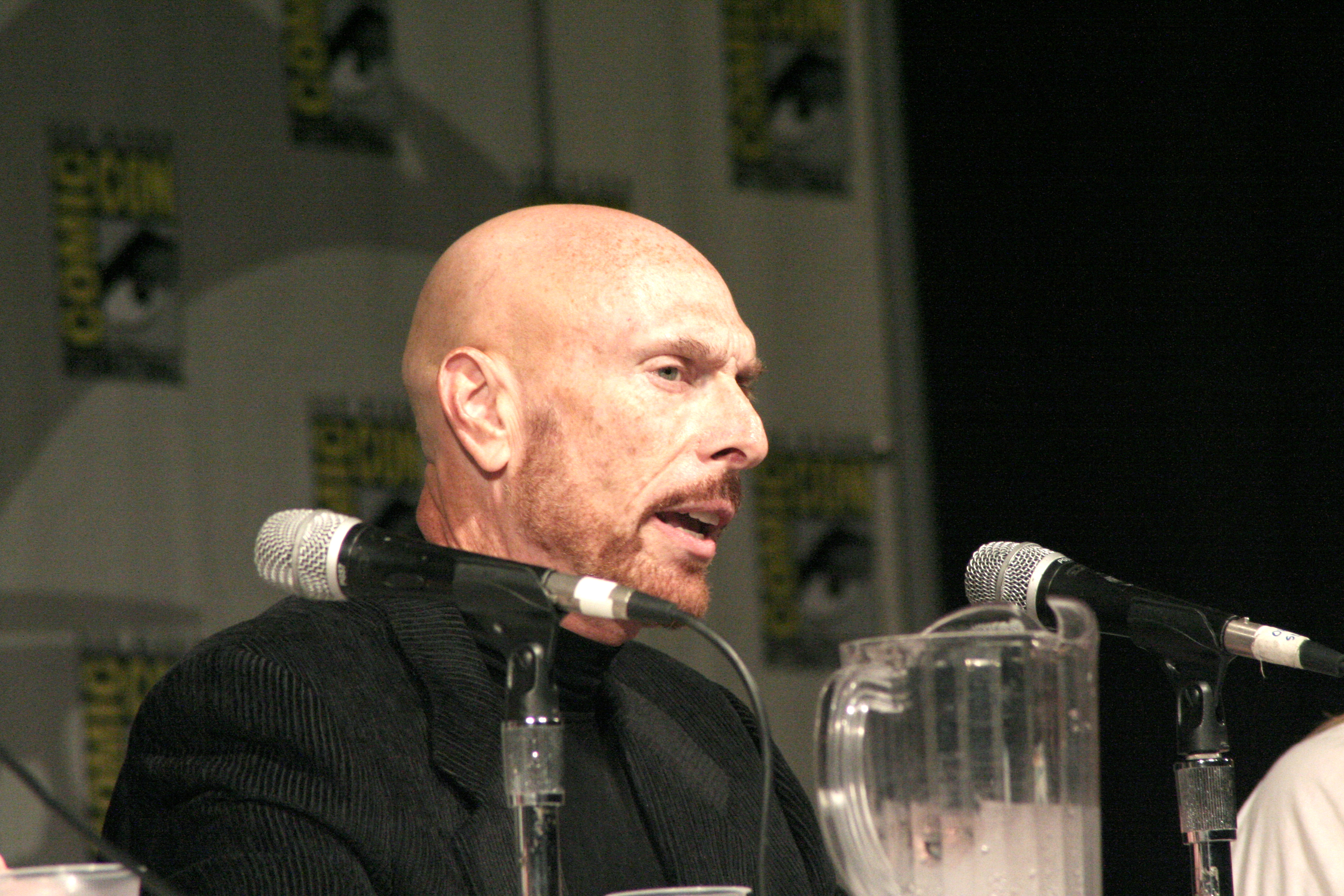The image captures author Terry Goodkind at what appears to be a panel at Comic-Con. The background features a repeating Comic-Con logo on a white wall. Goodkind, wearing a black jacket and a black shirt, is the focal point of the image. He has a shaved head and brown facial hair covering his jaw, chin, and upper lip. He is seated behind a table equipped with a microphone on a stand directly in front of him, a half-full pitcher of water to his right, and another microphone further down to the left. Goodkind appears to be speaking, as his mouth is open and he is gazing out towards the audience to the center right of the frame. A partial view of another individual’s shoulder is visible on the right edge of the photo.